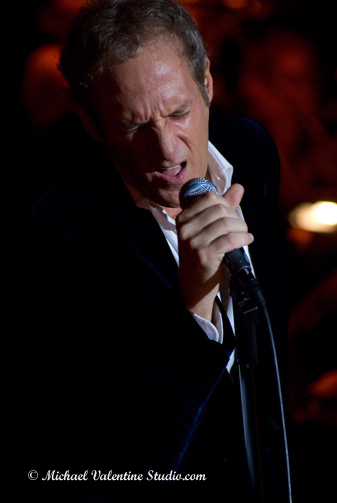The photograph captures a soulful moment of singer Michael Bolton, who is performing with his eyes closed, deeply immersed in his song. He is framed in a dark jacket and a white, open-collared shirt, his short hair a mix of brown and gray. Bolton holds a microphone in his right hand, the microphone connected by a black cord that dangles down. The microphone is attached to a stand. His expressive face, featuring visible sideburns, conveys the emotion of his performance. The backdrop is a blend of dark hues with prominent reddish tones and a faint yellow circle of light in the middle right, suggesting a nightclub-like atmosphere. In the bottom left corner, the image is marked with a copyright symbol and the text "michaelvalentinestudio.com" in small, white cursive script.